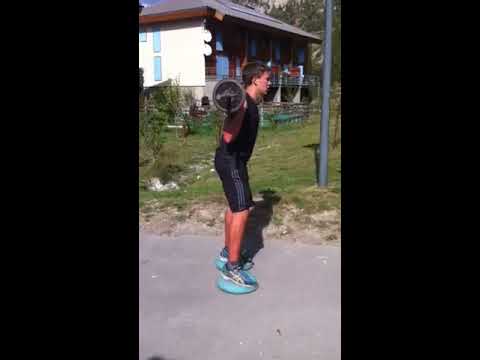The image features a young man working out, holding a barbell behind his head while standing on a paved surface, likely a sidewalk or piece of cement. He's dressed in a black shirt and black shorts adorned with silver or white stripes, and has on light bluish-green shoes with white accents. His stance suggests he's balancing on two unique pieces of equipment designed for stability training, described as plastic-based with a squishy, yoga-ball-like top. The setting is outdoors, with the mid-ground to his left showcasing some green grass that has bare spots. In the background stands a house with a brown roof and a yellow wall facing the camera, blue shutters, and minimally filled-out shrubs or bushes in the yard. A gray pole is visible in the upper mid-right section of the photo. The scene also includes a touch of visible sky above the house’s roof in the top left corner. The composition is bordered by two large blocks on either side, taking up about a quarter of the image each.